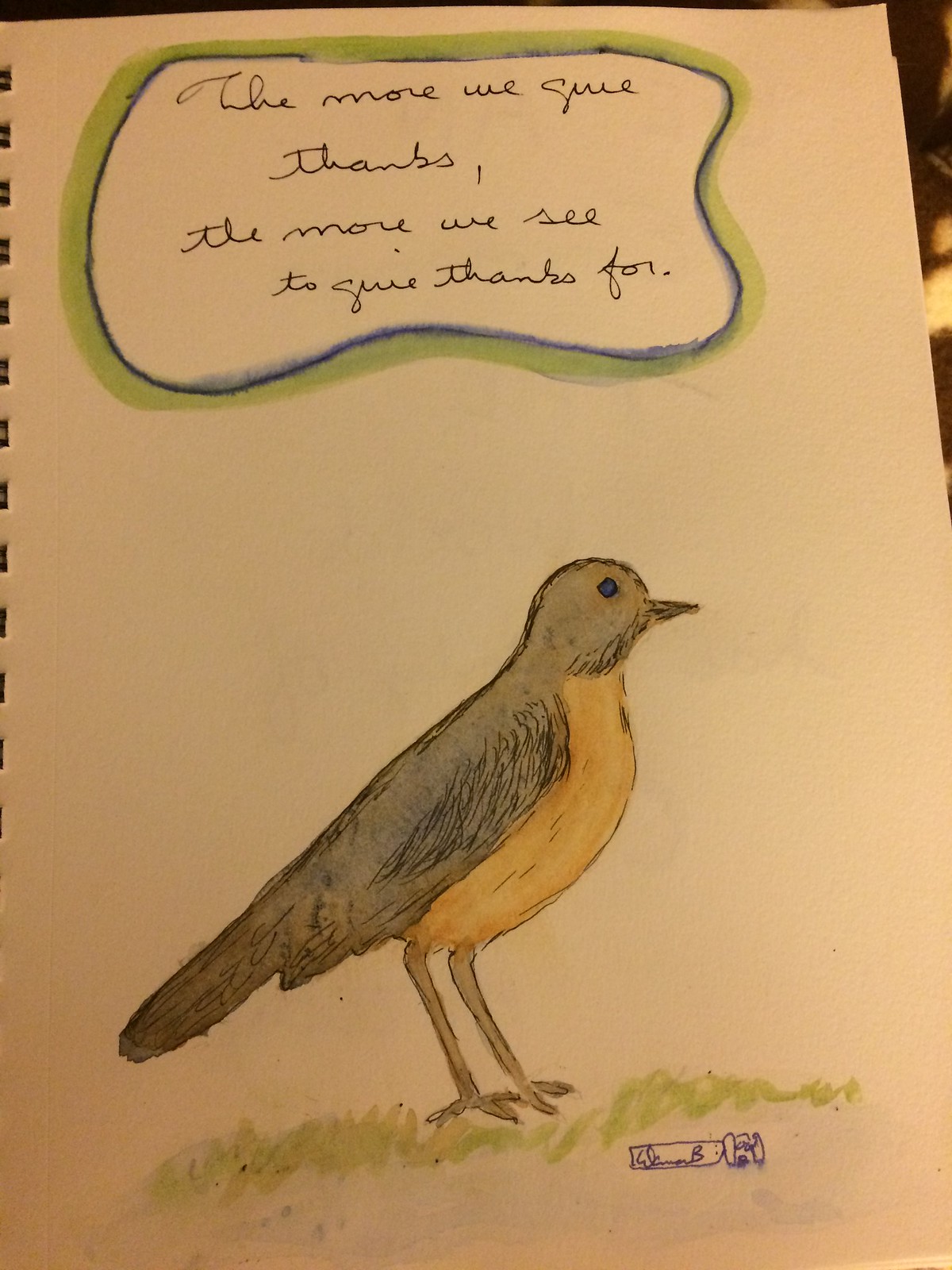This is a photograph of a hand-drawn card on white sketchbook paper, with visible wire spiraling on the left side binding. The card features a detailed drawing of a bird, likely a robin, portrayed in profile with distinctive attributes: a gray body, yellow belly, gray wings and legs, and black eyes and beak. The bird stands on a small patch of green grass, with a blue object faintly visible beneath it. Above the bird, there is an inspirational quote written in dark ballpoint pen cursive, reading "The more we give thanks, the more we seek to give thanks for." This text is encased in a blue quotation bubble bordered by a thicker green line. The mediums used for the artwork appear to be pen and watercolor, evidenced by some smudging where the water has slightly overrun the blue line around the quote. Below the bird, the artist has signed their name, which appears to be Elon B, followed by a small symbol. All these elements together suggest the thoughtful creation of an uplifting and artistic piece.